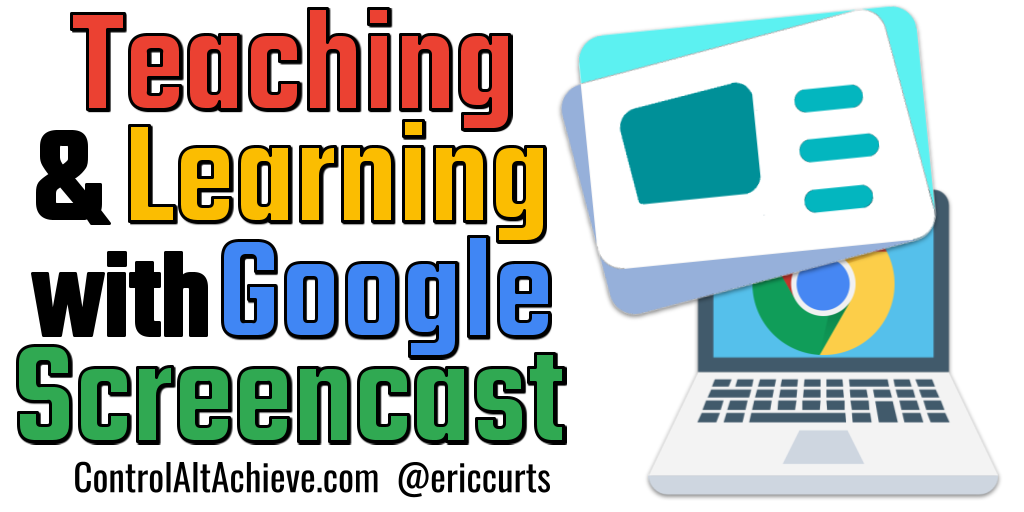This is a detailed digital drawing, serving as an advertisement for a learning course called "Teaching and Learning with Google Screencast." The background is plain white, bringing focus to the colorful elements of the design. On the right side, there is an illustration of a grey laptop with darker-colored buttons. Its screen is blue and prominently displays the Google Chrome logo. Positioned above the laptop are two squares: one light blue and one teal, each containing a white card in the center. On the left side of the image, five lines of text stand out in vibrant colors: "Teaching" in red, "&" in black, "Learning" in yellow, "With" in black, "Google" in blue, and "Screencast" in green. Beneath this colorful text, in black letters, it says "Control-Alt-Achieve.com Eric Kurtz." The advertisement is vividly colored with red, yellow, blue, green, and black, effectively highlighting the various elements of the course being promoted.